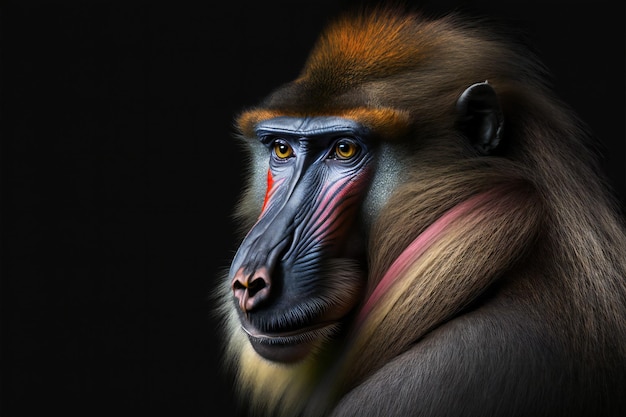The image showcases a majestic baboon with intricate detail and vibrant colors, set against a completely black background that emphasizes the subject. The baboon's face is a striking mix of bluish-gray, pink, and red hues, particularly highlighting his cheeks and nose. His expressive auburn eyes stare off into the distance, adding a sense of depth and contemplation. He has a bushy mane-like fur around his chin, similar to a lion's, and you can see his ear peeking through. The fur on his head is a stunning blend of brown, orange, yellow, and a hint of pink. It’s so vivid that you can see individual hair strands, making it appear almost too perfect, as if it could be an exceptionally well-taken photograph or an AI-generated image. The profile view captures part of his shoulders, with a distinct pink streak draping down, and the orange tufts of fur at the top of his head create a captivating contrast.